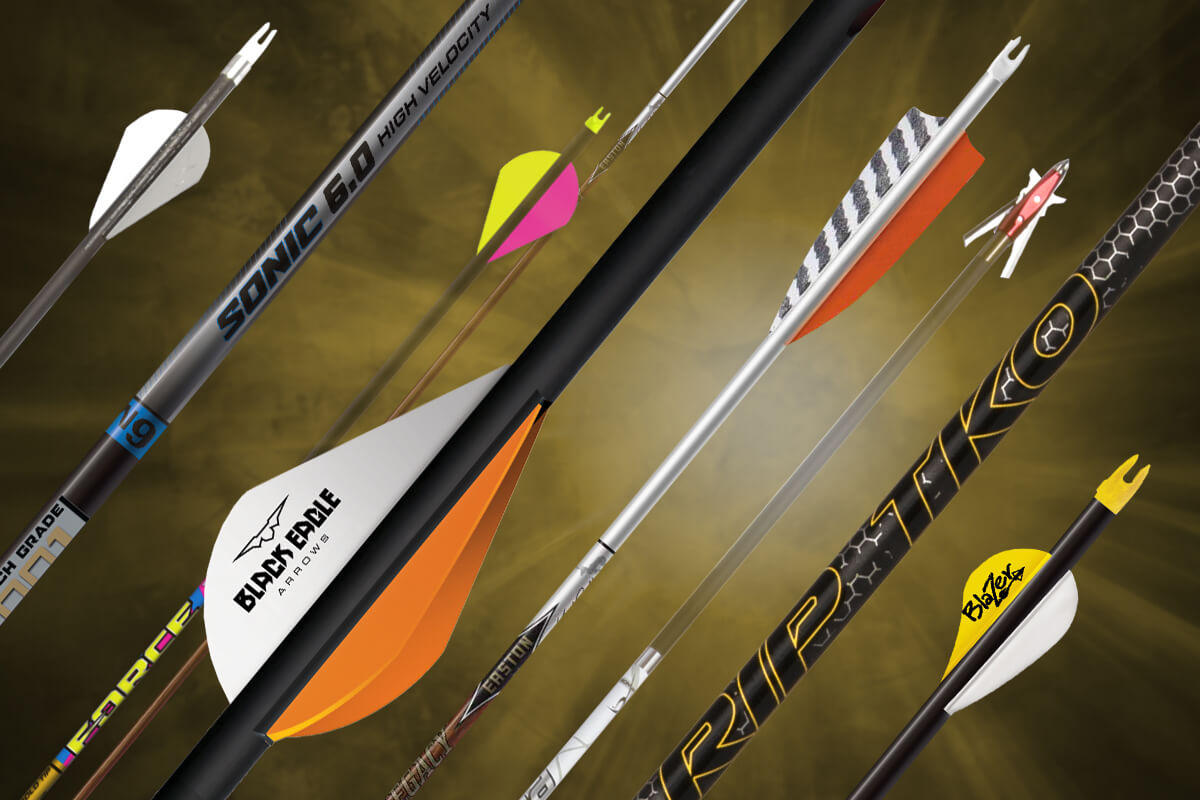The image showcases a dynamic composition of numerous darts and arrows, resembling those used in archery and dart games often found in bars. These projectiles are varied in both color and design, featuring handles and shafts in shades of silver, gray, black, orange, yellow, pink, and white. Each dart and arrow is marked with distinct logos, such as "Black Eagle," "Sonic 6.0 high-velocity," and "Blaze." The backdrop is an olive green and goldish sunburst gradient, radiating outward from just right of center, giving it a vibrant, almost solar appearance. All the arrows are aligned diagonally, pointing towards either the top right or bottom left, creating a unified and visually captivating effect. The meticulous detailing of the arrows includes plastic fletchings in neon and traditional colors, attaching to their sleek carbon or metal shafts.